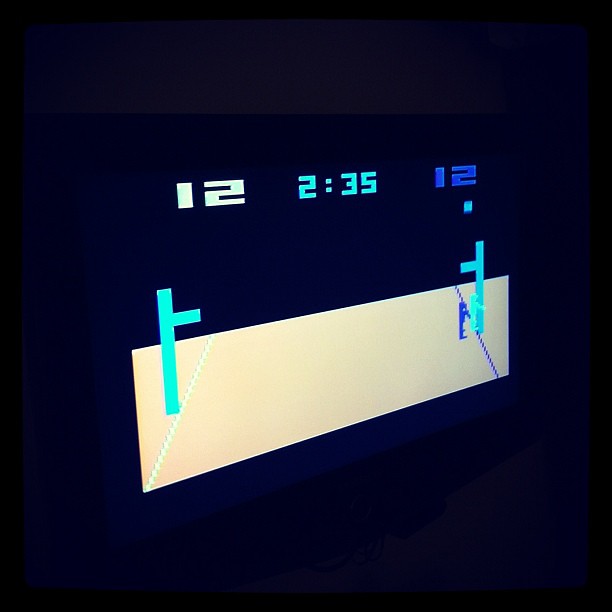This image features a predominantly black rectangular background. In the upper third of the black box, numbers are displayed in various shades of blue. Starting from the left, the number "12" is depicted in light blue, followed by a space. Next, in a teal blue hue, the numbers "2:35" are present, followed by another space. Finally, the number "12" appears again, this time in a darker blue color.

Beneath these numbers is a horizontally-oriented rectangle in a pinkish hue. Below this rectangle, two blue lines are drawn. These lines resemble the shape of the letter "F" - however, they are depicted differently. One line looks like a capital "F" with the top horizontal stroke missing, and the other line mirrors this shape but faces the opposite direction, making it appear as if the top portion of the "F" is missing on the inverted side.